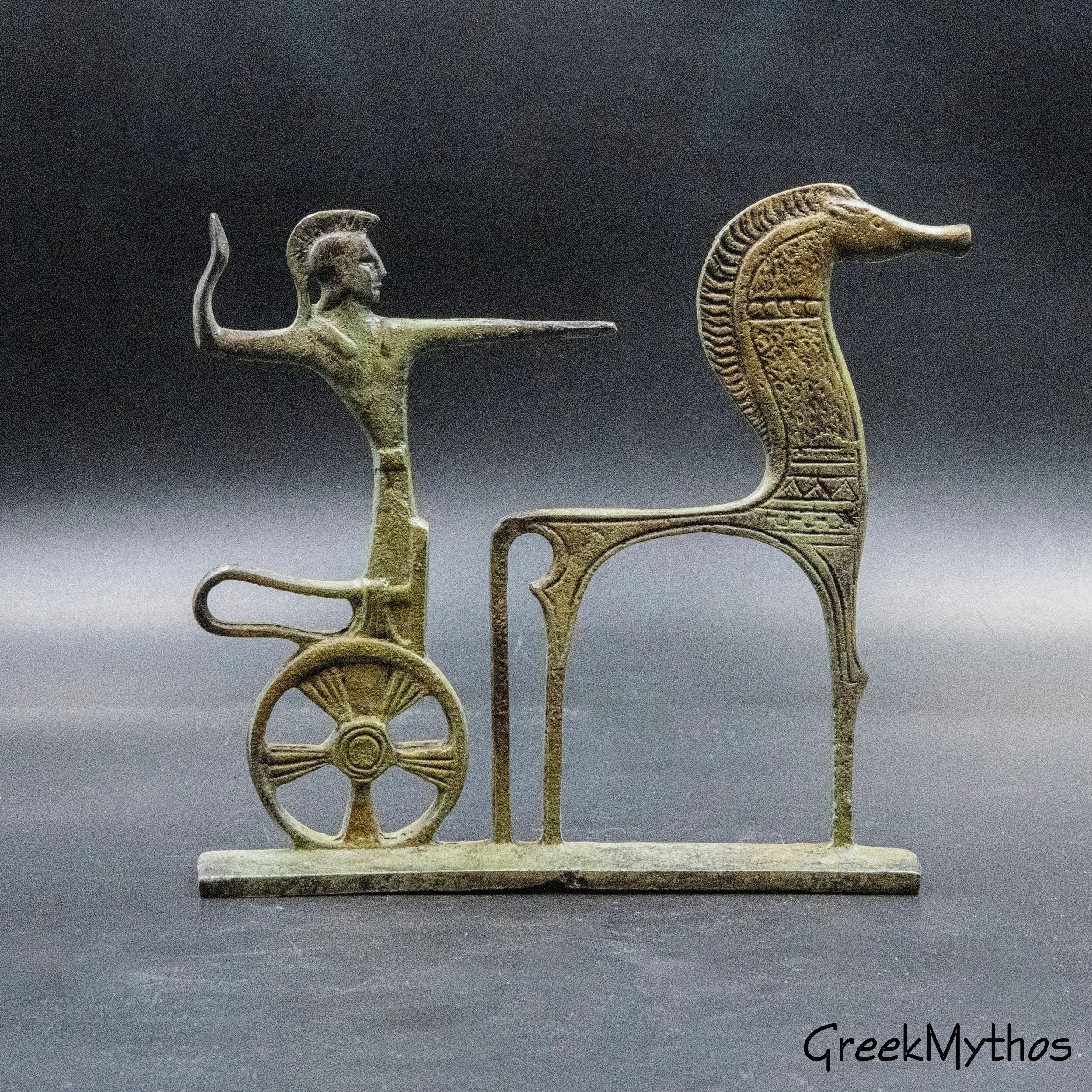The image is a detailed digital photograph of an antique metal statuette representing elements of Greek mythology. The central focus of the artwork is a horse-like creature, meticulously engraved with intricate patterns. To the right of the creature, a male figure, possibly a Greek warrior or mythological character, is depicted standing on a one-wheeled carriage. The figure's left arm is stretched out in front of him, while his right arm is raised upwards, as though holding something at bay. The statuette is crafted from a blend of metals, bearing colors of black, bronze, gray, and moss green. The bottom right corner of the image features the inscription "Greek mythos," alluding to its mythological theme. The background of the photograph is a subdued gray, enhancing the prominence and detail of the statuette.